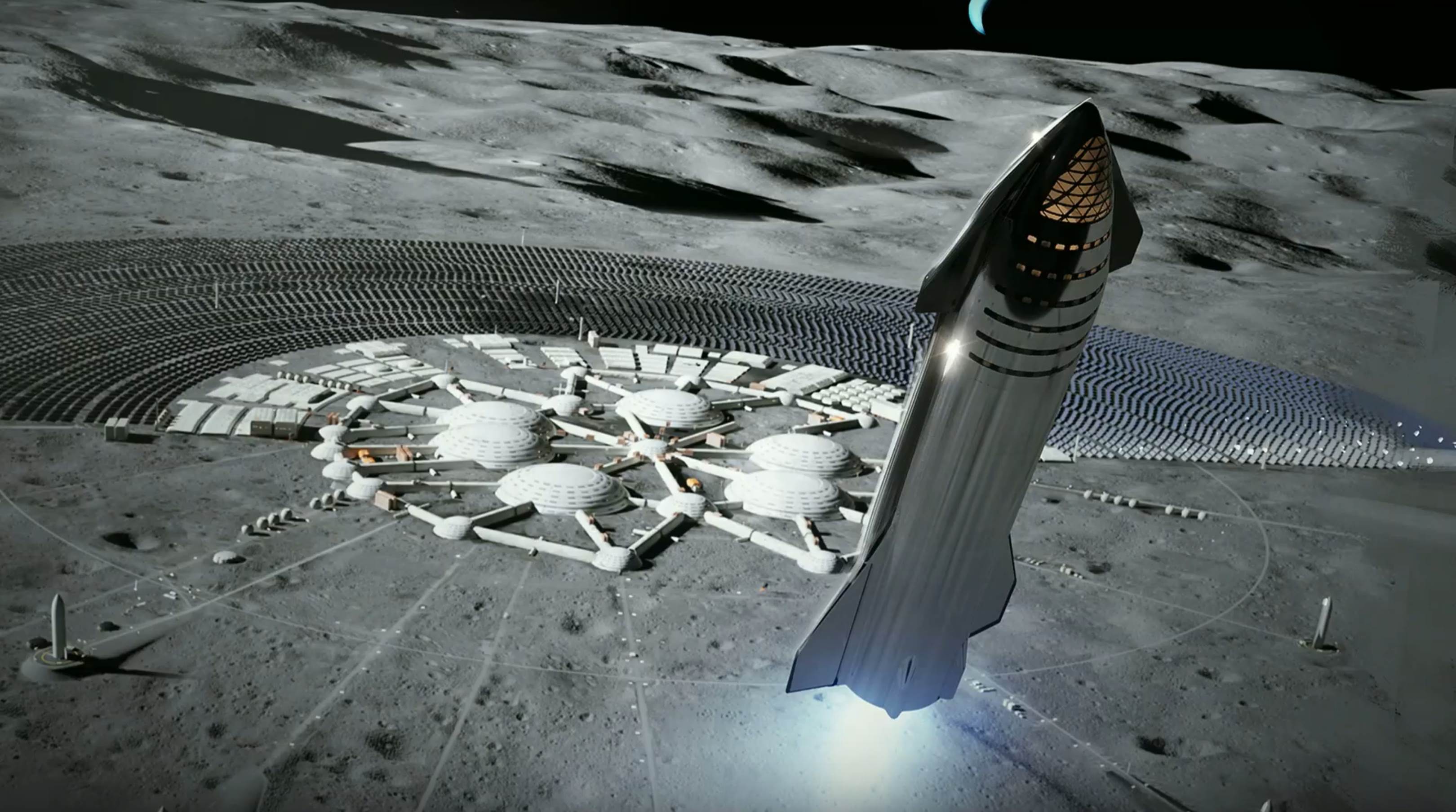In this digitally created image, a sleek and chrome SpaceX spaceship, resembling a phallus and designed for vertical landing, is prominently positioned in the foreground. The vessel appears to be either landing on or taking off from a moon-like surface, characterized by a white and gray, crispy texture typical of lunar landscapes. In the background, there is a large, intricate space station comprising six interconnected dome-shaped pods, resembling white frisbees connected by tubes that look like PVC pipes. Arrayed behind these domes is a semicircle of solar panels. The environment's backdrop displays a stark black atmosphere, accentuated by a crescent shape, adding to the outer space setting. This scene, depicted entirely in black and white, captures a moment of advanced human space exploration and colonization efforts on the moon.